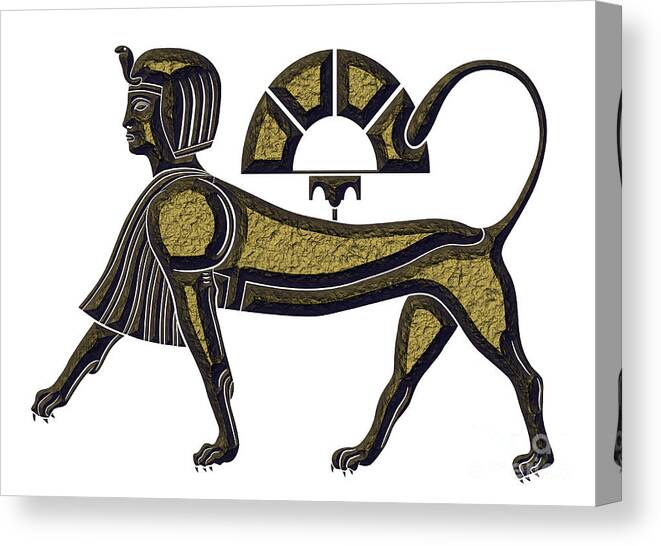This image depicts a digitally generated piece of artwork displayed on a three-dimensional, white rectangular canvas. The focal point is a surreal and intricately detailed hybrid figure, combining the head of a human with the four-legged body of a large feline. The style evokes a blend of hieroglyphic artistry and modern digital intricacy. The color palette features gold, black, white, and brown, with shadows adding depth to the golden hues. The human head is adorned with an Egyptian-style helmet, featuring a distinctive cobra-like snake emerging from its front, enhancing the mythical and ancient aura of the artwork.